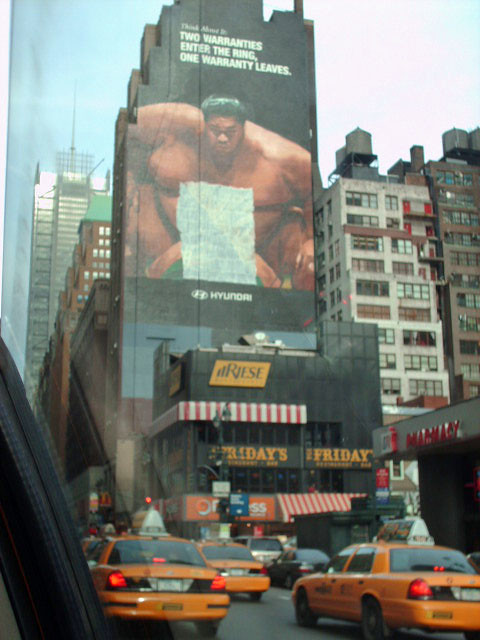The image depicts a large, vibrant billboard that appears to be situated in a bustling urban area similar to Times Square in New York City. The billboard features a dramatic and humorous illustration of two larger-than-life sumo wrestlers in a wrestling ring. The text at the top of the billboard, although somewhat difficult to read, states: "Two Variantes enter the ring. One Variante leaves." This tagline plays on the iconic imagery of sumo wrestling to humorously advertise car warranties. Beneath the sumo wrestlers, the logo and name of Hyundai are prominently displayed, indicating that this is an advertisement for Hyundai car warranties. Adding to the lively scene, the street below is filled with the characteristic yellow cabs of New York City, and a TGI Fridays restaurant is visible, further suggesting the location is likely Times Square.